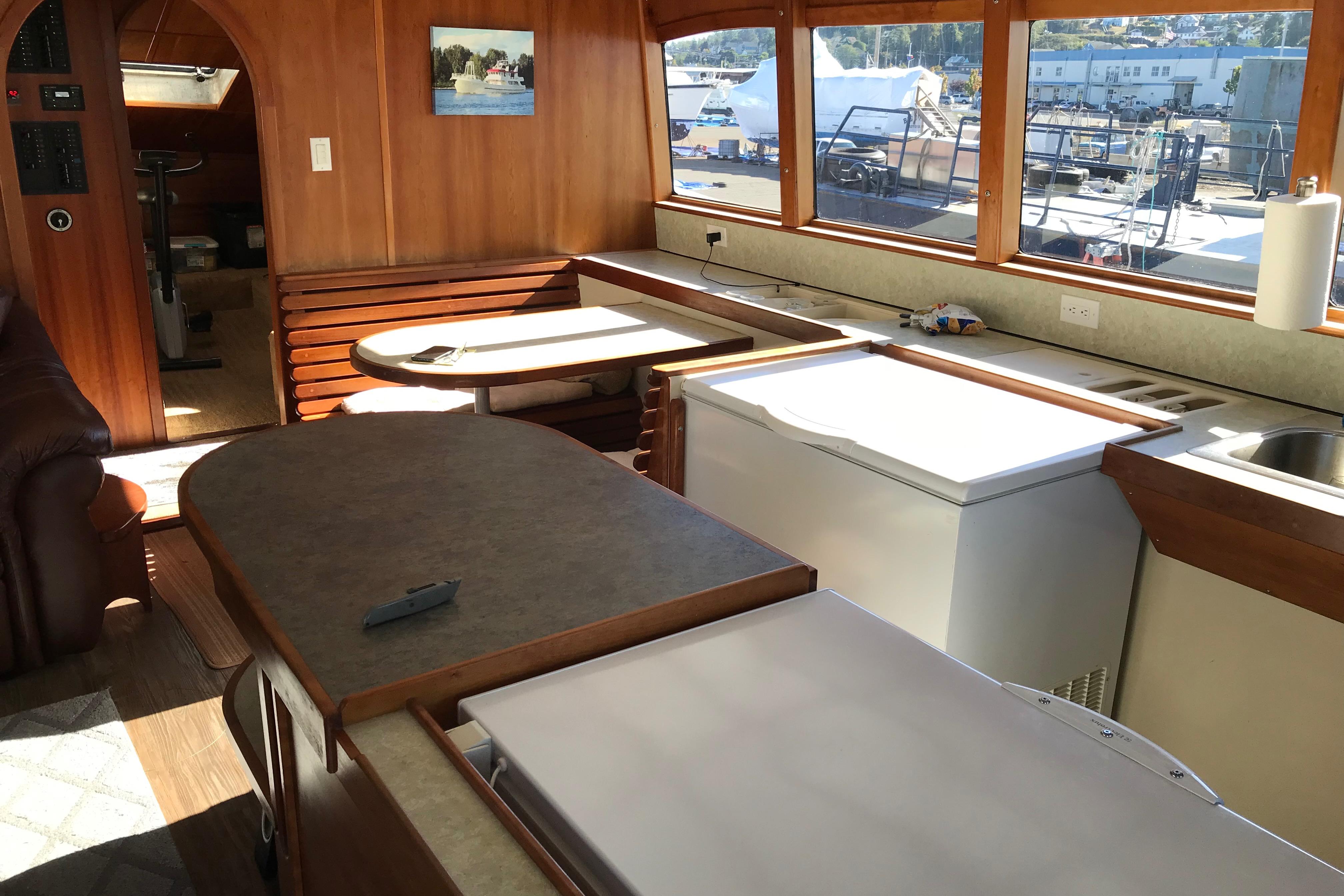The image depicts a cozy interior space, likely the kitchen area of an RV or boat. Dominating the center of the room is a compact kitchen island featuring a brown and white table perfect for food preparation. Adjacent to this island is a freezer, while another freezer and a sink with a preparation strip are situated on the opposite wall, which also boasts several sockets for electrical outlets.

The room is framed by wood laminate paneling on the walls and geometric-patterned laminate flooring. In the upper left corner of the scene, a small nook with brown bench seats around a white tabletop provides a cozy seating or dining area reminiscent of camper interiors.

To the upper right, three horizontal grid-style windows trimmed in medium wood offer a view of what appears to be an industrial-looking shipyard or dockyard. Visible through the windows are elements like docks, a black fence lining a narrow walkway, and distant buildings that suggest the setting is by a waterfront or marina. The room is bathed in light from these windows, adding to its warm, inviting atmosphere.